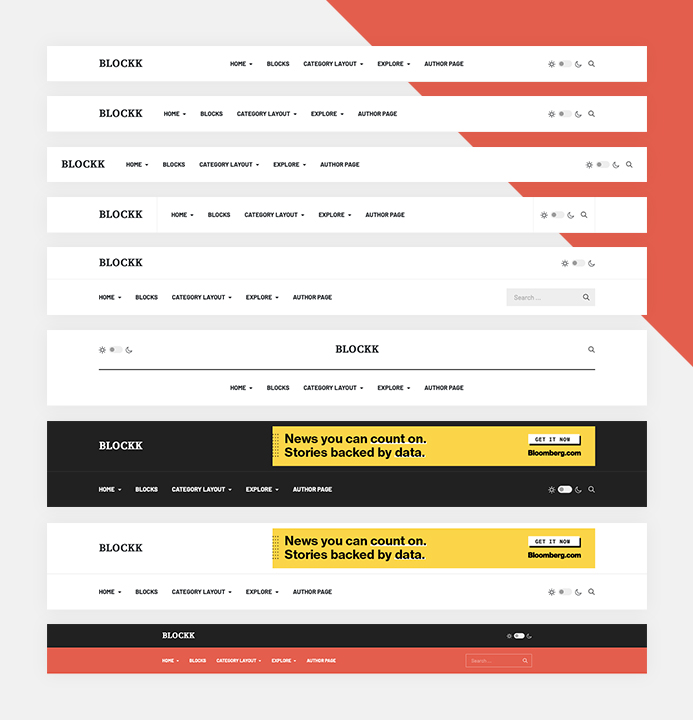This image displays various layouts for potential news articles. Featured prominently at the bottom is the word "block," spelled out as "B-L-O-C-K-K" in a descending vertical orientation. The design repeats the term "block" multiple times across the image. 

The interface offers options for additional blocks, a category layout, an exploration of an author page, and multiple icons including a search icon, numbered one through five. Below these elements, the pattern of "block" and search icons reappears, followed by prompts for more blocks, a category layout, and an author page exploration, all in a list format.

In the middle section, "blocks" are highlighted in black, and at the bottom of the image, navigation options are displayed in white, including home, blocks, category layout, and author page exploration.

The phrase "news you can count on, stories backed by data, bloomsburg.com" is presented twice—first on a black background and then on a white background underneath. The repeated navigation options at the bottom reiterate home, blocks, category layout, and explore author page.